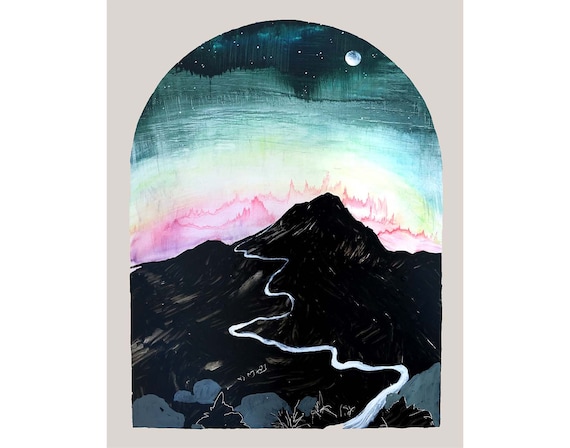This image is a multi-color artistic piece devoid of borders, set against a light purple background. The painting itself is vertically rectangular with an arched top, resembling the shape of a tombstone or bullet. It depicts an abstract outdoor landscape with a prominent dark mountain in black and brown hues, without any snow. A white, wavy line, which could represent either a stream or a road, begins at the base of the mountain, emanating from a low pass to the left and moving toward the center. Above the mountain, the sky bursts into a cascade of vibrant colors, including reds, blues, yellows, pinks, and dark green, creating an abstract splash. The sky transitions to black at the top, dotted with a few stars and a full moon positioned in the upper right area. The overall composition suggests a mix of watercolor and abstract styles, merging the terrestrial with celestial elements in a vividly imaginative scene.